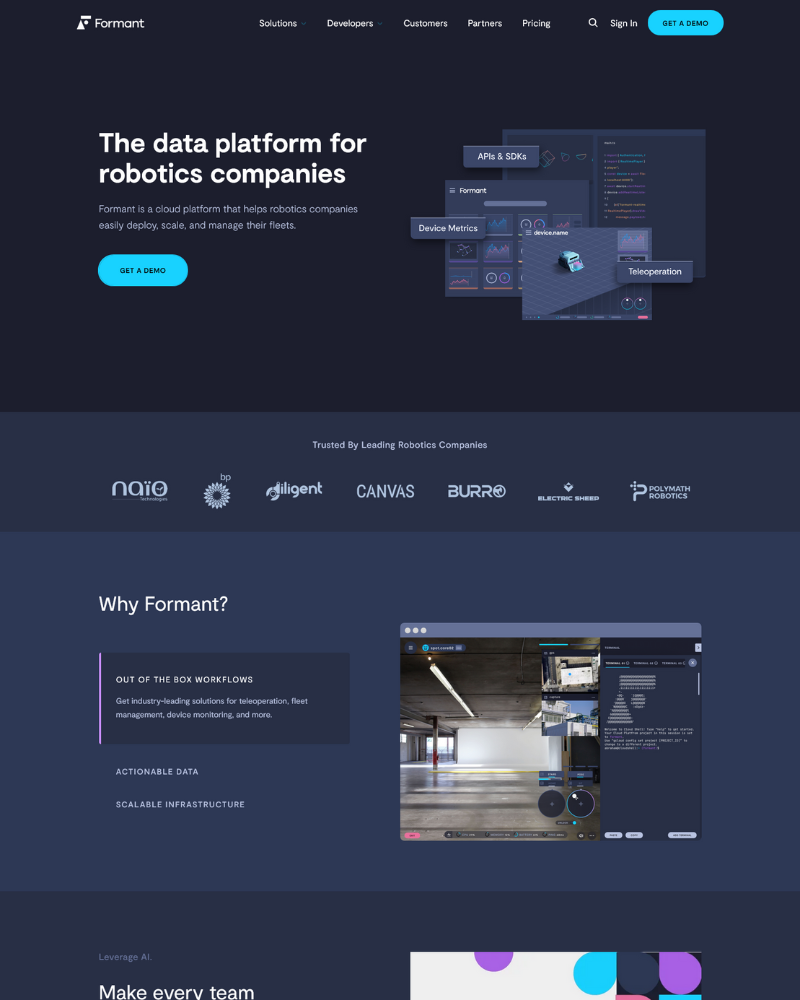The screenshot captures a webpage for a company named Formont, which features a dark to light blue gradient background. At the top left corner, the company name "Formont" is prominently displayed. Adjacent to it, a navigation bar provides links to "Solutions," "Developers," "Customers," "Partners," and "Pricing," along with a magnifying glass icon for search functionality. To the right of the navigation bar, there are buttons labeled "Sign In" and "Get a Demo," with the latter presented in a distinctive blue oval shape.

Dominating the central area of the screenshot, large white letters announce "The Data Platform for Robotics Companies." To the right of this text, a series of images resembling computer screenshots are displayed. Beneath this section, another "Get a Demo" button is visible in bright blue.

In the lower half of the image, the headline "Why Formont" introduces several key features of the platform. Text below this headline highlights "Out-of-the-Box Workflows" and advertises solutions for "Teleoperation," "Fleet Management," "Device Monitoring," and other functionalities. Accompanying this text on the right is a picture of what appears to be an empty concrete warehouse. At the very bottom right, a small white rectangular box is shown, adorned with purple and blue dot designs, adding a touch of graphic detail to the page.